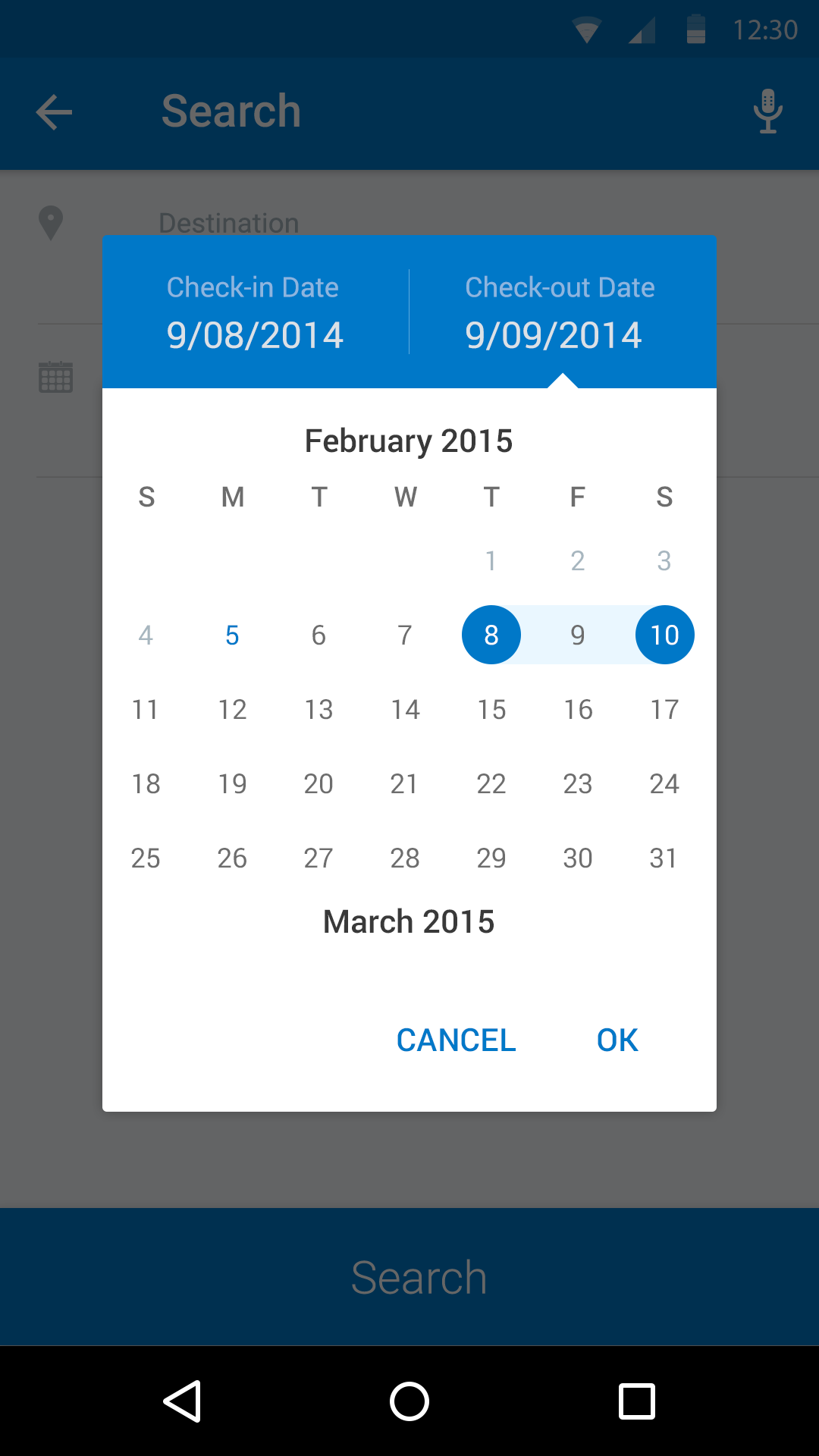This detailed caption provides an extensive description of a screenshot taken from a mobile phone screen displaying a hotel booking interface:

---

A screenshot of a mobile phone screen displays a hotel booking interface that is predominantly themed in shades of blue and gray. At the top of the screen, a dark blue status bar shows key indicators: a strong Wi-Fi signal, full cellular signal strength, high battery levels, and the current time of 12:30. Below this, a lighter blue navigation bar contains a white left arrow labeled "Search," and next to it, a white microphone icon, indicating voice search functionality.

In a lighter gray text, there is an input field marked "Destination," accompanied by a pin icon suggesting location input and a calendar icon next to it. Towards the bottom, a darker blue search box is prominently displayed with the word "Search" written in light gray.

The bottommost part of the screen is a black navigation bar that includes three icons: a solid left-pointing triangle (back), a hollow circle (home), and a hollow square (recent apps).

Central to the screenshot, dominating the middle of the screen, is the booking information showing the check-in and check-out dates in blue and white text: "Check-in Date: 9-8-2014" and "Check-out Date: 9-9-2014". Below this, a white calendar box for February 2015 displays the days of the week (SMTWTFS) at the top, followed by the numbered days of the month. Adjacent to it, there is also part of the March 2015 calendar visible.

Finally, two functional buttons are positioned at the bottom of the calendar: "Cancel" in blue text on the left, and "OK" in blue text on the right, allowing the user to either proceed or discard the date selection.